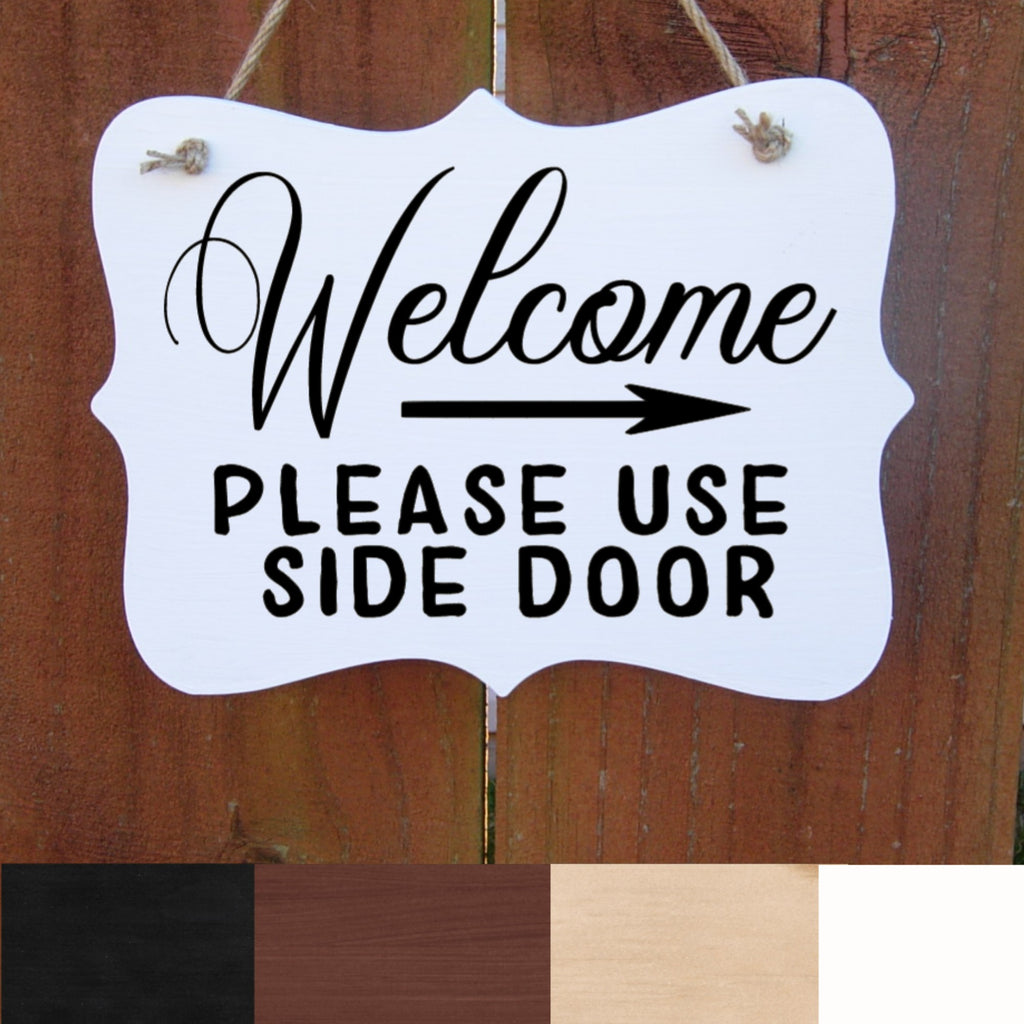This image likely from Amazon depicts a white, roughly rectangular welcome sign with stylized, curved edges and points in the middle of each side. The sign, which is supported by a piece of twine knotted through holes at the top, features black text in cursive reading "Welcome," accompanied by a right-pointing arrow. Below, in non-cursive text, it instructs "please use side door." The sign is displayed against a brown wooden surface, which could be a door or fence, showing visible wood grain and a vertical seam. At the bottom of the image are color swatches in black, dark brown, and a light tan, suggesting these are color options for the same sign.